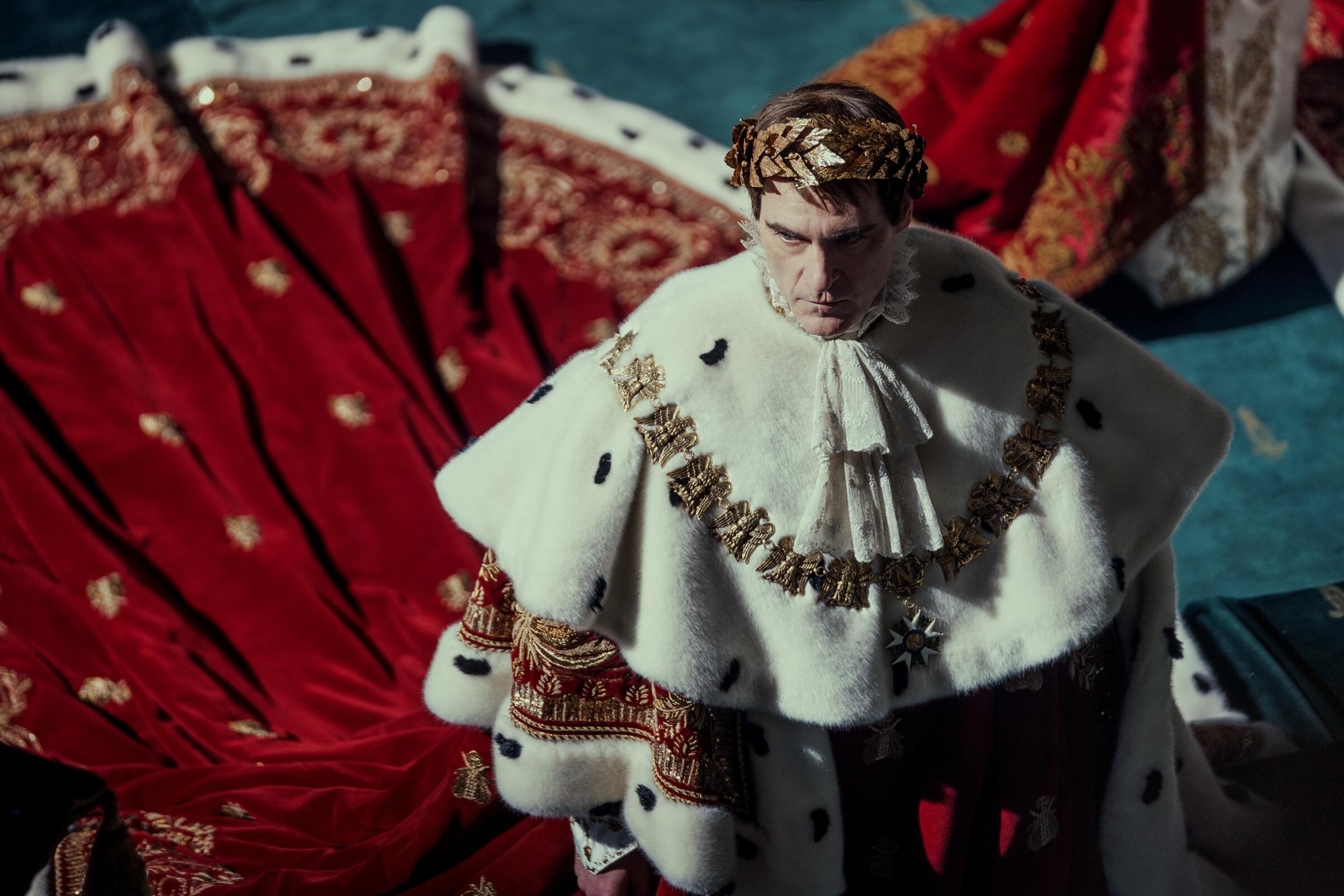In this professional-looking image, we are looking down at a distinguished figure dressed in regal attire, likely depicting Joaquin Phoenix as Caesar from the movie *Julius Caesar*. The scene is shot from a downward angle, accentuating the character's age and stern expression. He is adorned in an elaborate outfit that includes a white long cloth and an extensive train resembling a wedding train, which extends about 8 feet behind him. The train is rich red with intricate gold designs and white trim along the edges. Additionally, he wears a crown of leaves, enhancing his royal appearance. The background features a blue floor and another figure dressed in red with gold accents, contributing to the luxurious and authoritative atmosphere of the image.